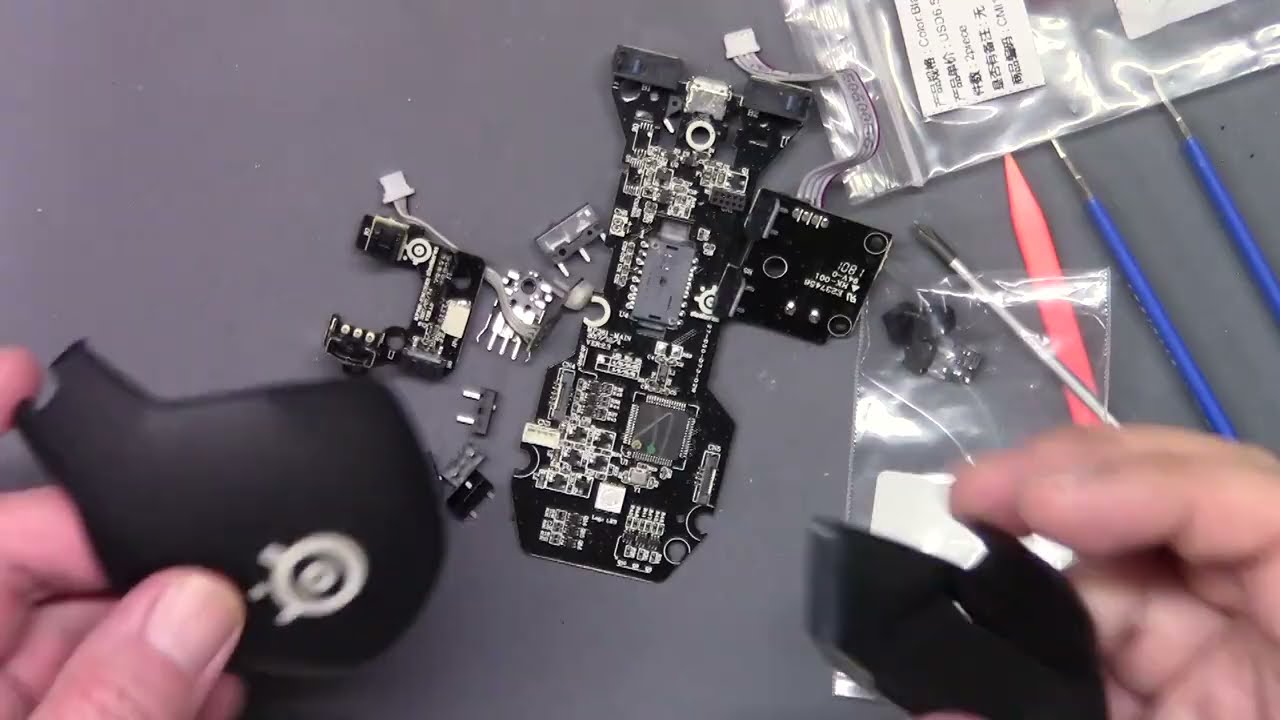The image depicts a work area on a dark gray table or counter, with disassembled computer components spread across it. At the center is a prominently placed, rectangular black motherboard or electronics board with numerous small, intricate gray compartments. Surrounding this central piece are various additional electronic items, including smaller boards and cables that appear to be intended for soldering or assembly.

In the upper left-hand corner, there is a small Ziploc baggie with a label containing various symbols. The lower left-hand corner reveals part of a person's hand, holding a black object with a distinctive white SteelSeries logo, characterized by two concentric circles with extensions on the top and left. The lower right-hand corner shows the other hand holding another small black object, which seems to be part of the assembly process. These hands hold pieces of what is likely the shell of a mouse, specifically a SteelSeries mouse.

Adjacent to the person's right hand, just below it, there is another elongated Ziploc baggie, and the upper right-hand side of the image shows three sharp tools with blue handles and silver tips. These tools are arranged neatly beside yet another clear plastic bag with a white sticker on it. The overall scene suggests a meticulous assembly or repair station, highlighting an array of components and tools associated with building or fixing digital chips—possibly for a computer mouse.